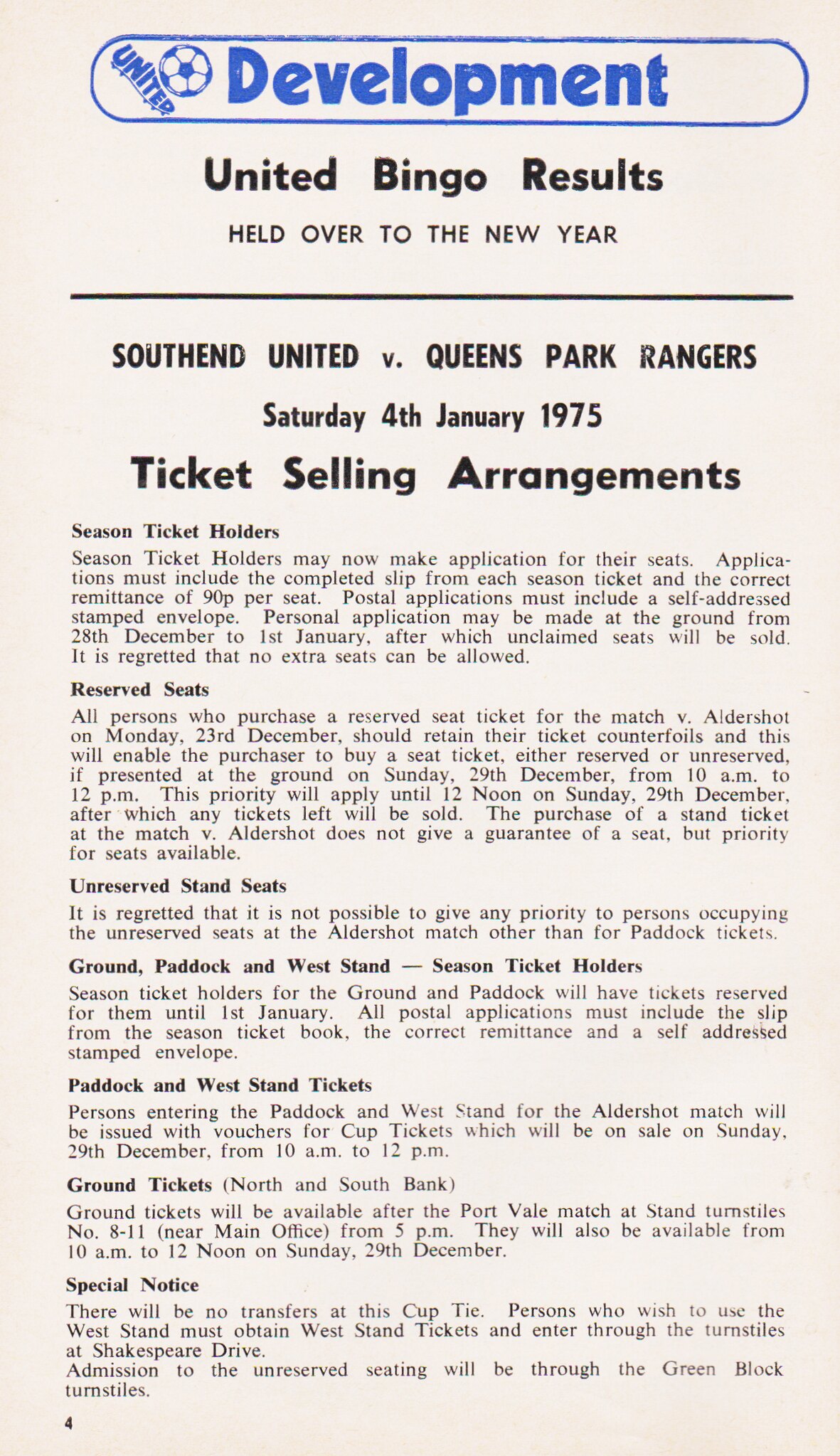The image is a vertically aligned rectangular flyer on a white sheet of paper, distinguished by a white and blue-themed design. At the top, it prominently features the word "Development" in bold blue letters, enclosed by a line, and is accompanied by a blue and white soccer ball image on the left, with the word "United" printed diagonally across it. Directly below in black text, it reads "United Bingo Results" followed by "held over to the New Year." 

Beneath a separating horizontal line, the flyer details "South End United vs. Queens Park Rangers" with the event date "Saturday 4th, January 1975." Below this, a headline "Ticket Selling Arrangements" introduces several sections of text, each with its own heading. The first heading reads "Season Ticket Holders," followed by several lines of text. The next section is titled "Reserved Seats" with a corresponding block of text, then "Unreserved Stand Seats" with two lines of text. Further down, headings like "Ground, Paddock, and West Stand - Season Ticket Holders," "Paddock and West Stand Tickets," and "Ground Tickets (North and South Bank)" each precede their respective text blocks. The last heading, "Special Notice," is paired with additional details. In the bottom left-hand corner of the flyer, the number "4" indicates the page number.

The text throughout the flyer is black and aligned in a justified format, making it clear and readable.